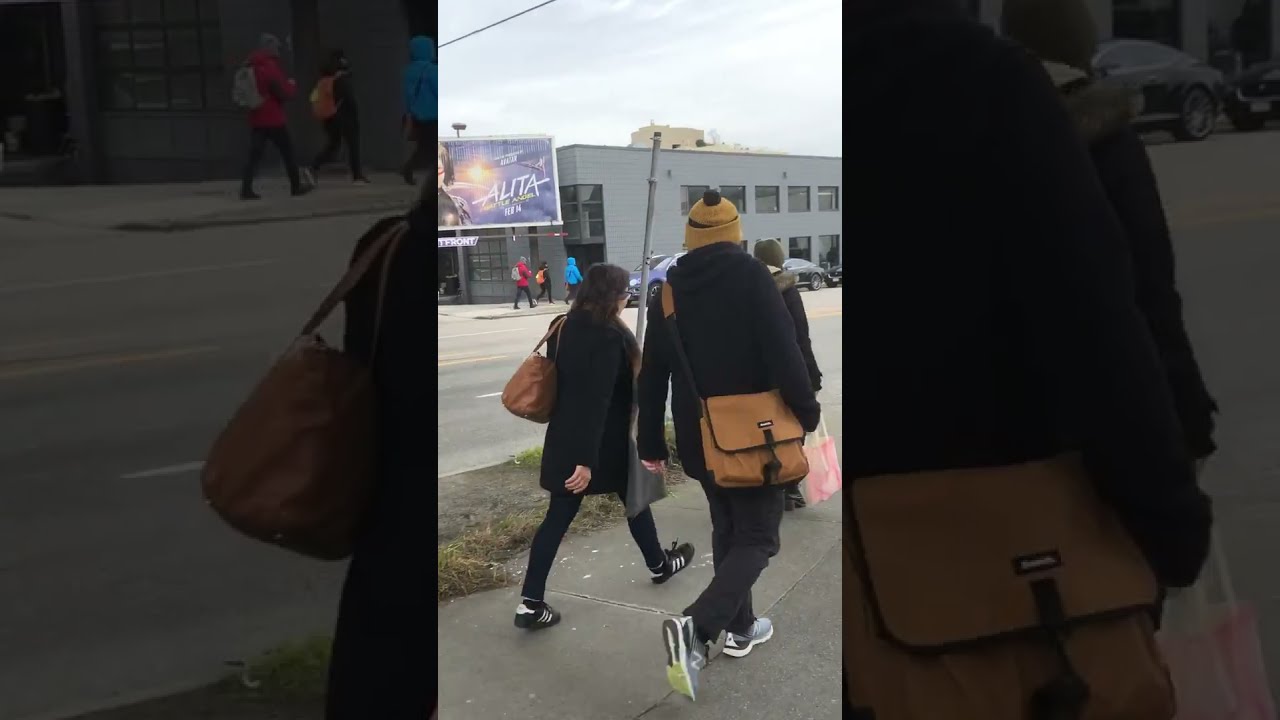In the center panel of a triptych, flanked by black panels on either side, the photograph captures a detailed street scene featuring two men walking on a city sidewalk. The man closer to the camera wears a gray overcoat, black scarf, gray stocking cap, and dark gray pants, carrying a black bag slung over his shoulder. Beside him, slightly ahead, walks another man with a darker complexion, donning a red stocking cap, black gloves, black jacket, and blue jeans. Both are heading to the right of the image. The sidewalk they tread is bordered by patches of overgrown grass when you look near the left edge, where a small sign is also visible. In the background, the scene unfolds with a glimpse of a city street lined with utility poles, power lines, and various buildings. Further back, a billboard featuring a woman stands against a gray, overcast sky, adding depth to the urban setting.